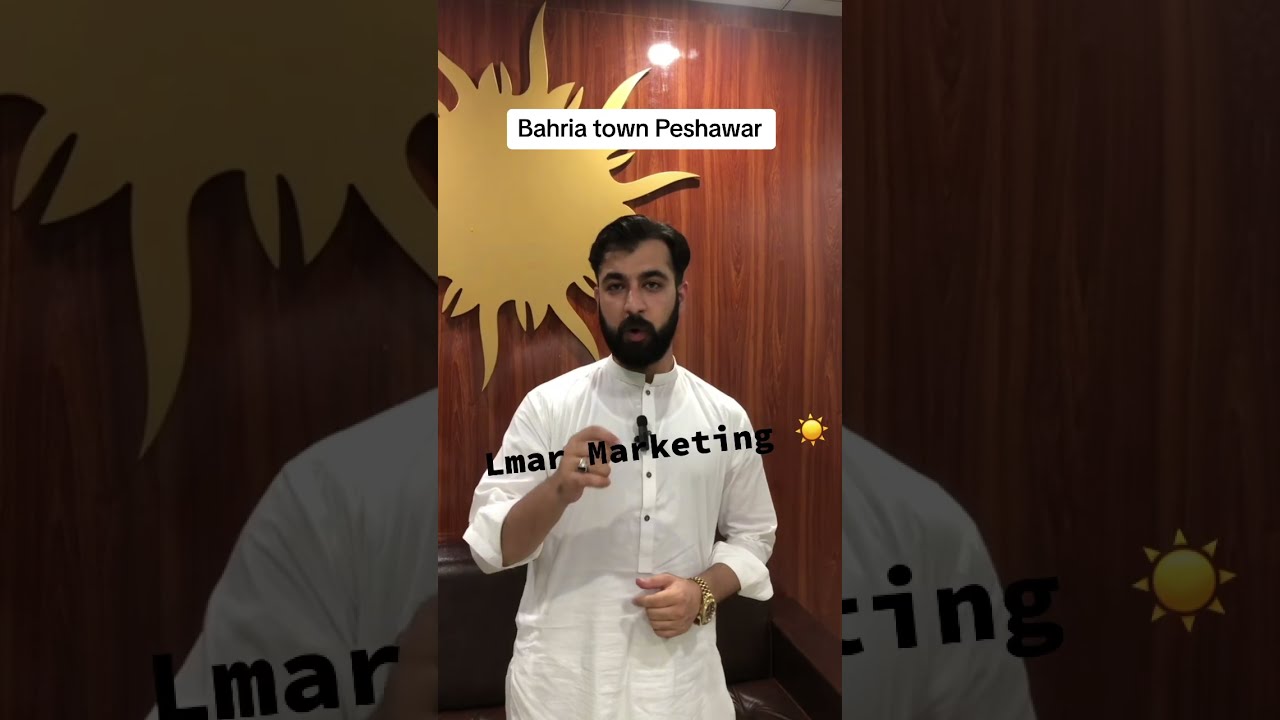The image is a screenshot of a social media page, likely TikTok or Instagram. It features an Indian or Pakistani man with brown skin, black hair, a full beard, and a mustache. He’s wearing a white button-up shirt with rolled-up sleeves, a gold wristwatch, and a golden ring on his right hand’s fourth finger. The man is standing against a dark brown wooden wall with a yellow sun or star design over his left shoulder. Text at the top of the image reads "Baria Town Peshawar" in black with a white background, and across his chest, in black text, it reads "Lamar Marketing" with a sun emoji. This appears to be a social media advertisement.